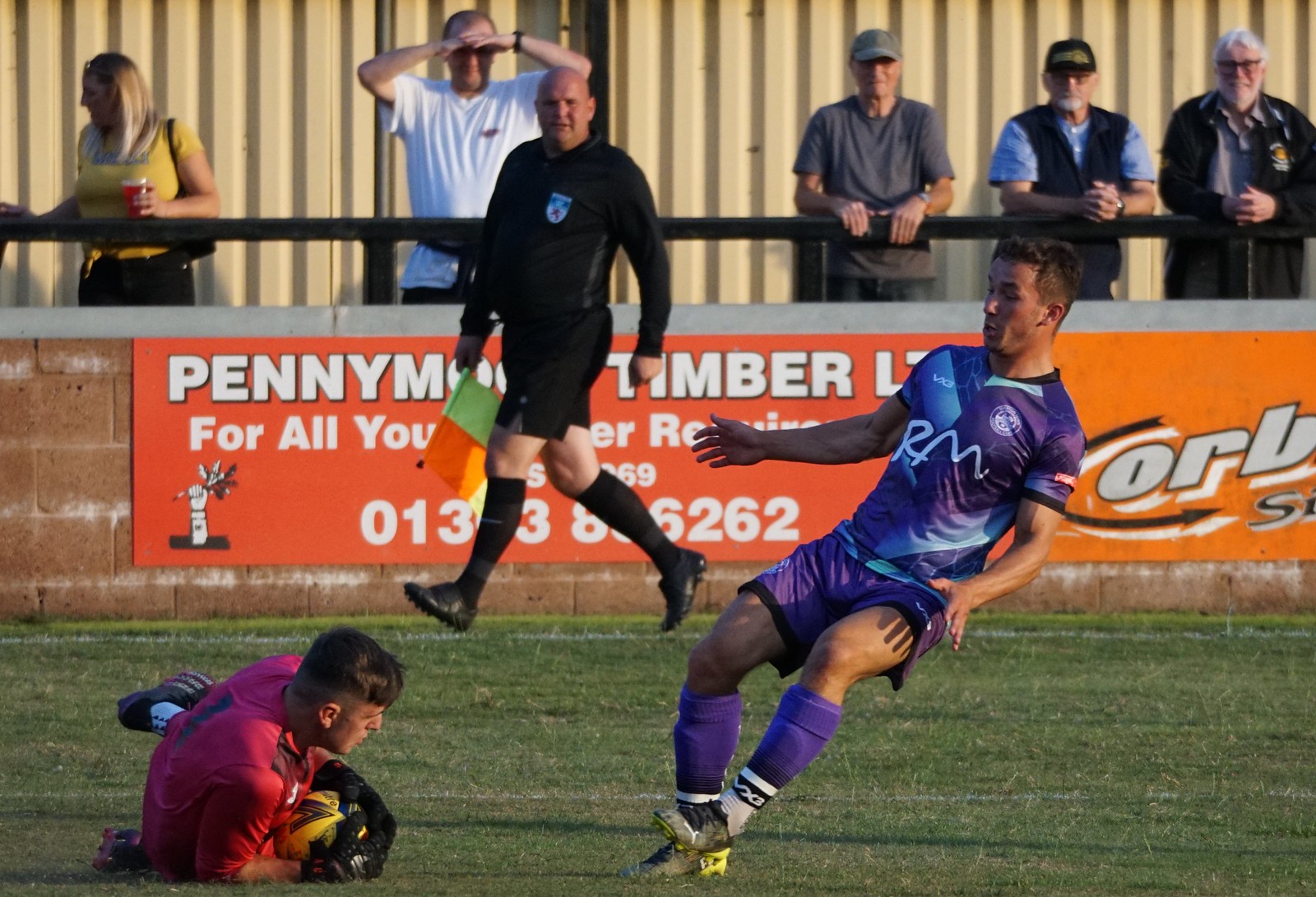In this lively outdoor soccer match, the image captures a dramatic moment as a player in a purple and blue uniform with knee-high socks and cleats slides toward another player in a red uniform, who is on the ground holding the ball. They are playing on a green turf field, marked with white chalk lines. The sliding player's intent and the fallen player's grip on the ball form the focal point of this intense scene. 

Supporting the action, a referee in black shorts and a black top, holding a red, orange, and green flag, is approaching the players. The background features a half-brick wall with a bold, two-toned orange advertisement reading "Panny M.O. Timber Limited for all year," accompanied by a phone number. The vibrant colors of the ad juxtapose against the backdrop. Further back, an assortment of spectators, four men and one woman, watch the game intently from behind a metal rail. Some of them have their hands on their heads, engrossed in the unfolding match, while others lean casually against the rail. The scene is capped off with a bright awning over the spectator area, highlighting the communal excitement and engagement in the game.